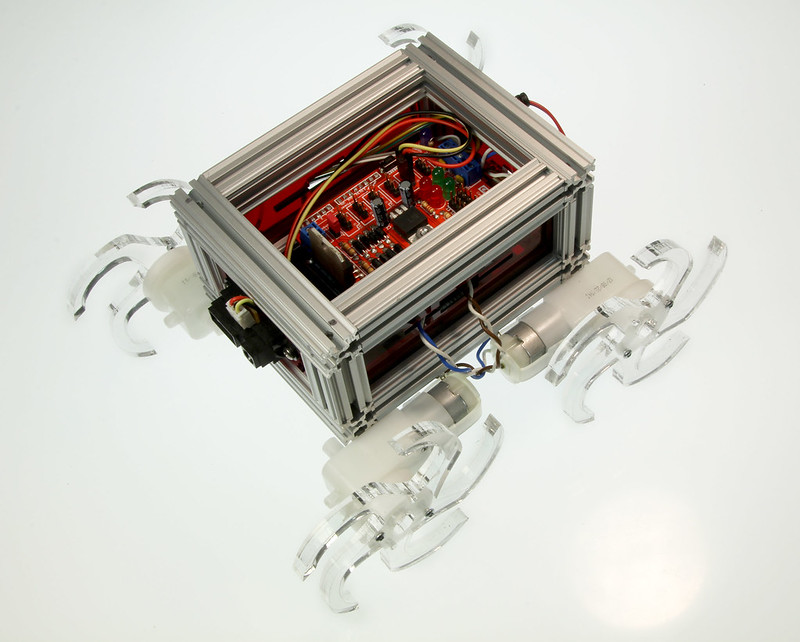The image showcases a close-up of a rectangular, Unistrut-framed robotic contraption against a white background. Within the open frame, a red PLC board is visible, surrounded by a complex network of wires, switches, fuses, and various electronic components, including sensors and relays. Secured to the four corners of the frame, transparent wheels with five curved, hook-like spokes are clearly seen. These wheels, resembling a fan or claw, are connected to motors by wires threading back into the main assembly, highlighting an intricate and detailed piece of machinery.